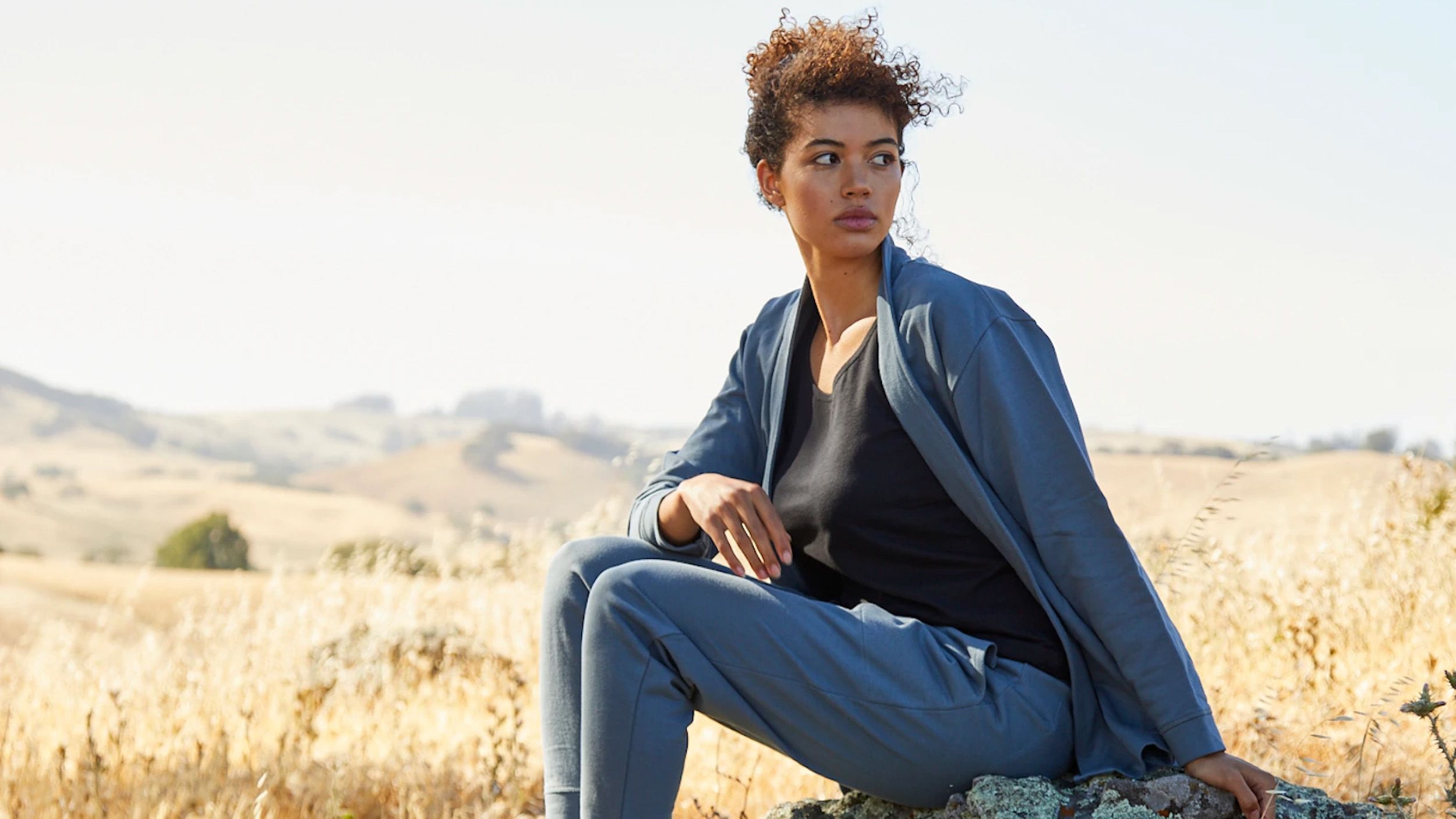In this captivating outdoor photograph, a young African-American woman in her twenties is the focal point, posing gracefully on a gray rock situated in the lower right corner of the image. The woman is dressed in a coordinated ensemble of a light blue-gray jacket and matching pants, with a loosely fitted black tank top underneath. Her auburn-brown curly hair is elegantly pulled up into an updo, accentuating her delicate features. She sits facing the left but turns her head to gaze over her left shoulder into the distance, with her right elbow resting on her right knee and her right hand dangling in front of her. Her left arm is positioned behind her on the rock, aiding her balance.

The backdrop, deliberately blurred to highlight her presence, reveals a vast, golden-hued field reminiscent of a wheat or savanna landscape. The field stretches out to meet a low-lying mountain range or hills in the far distance. Scattered within this serene expanse are a few scrubby trees, larger rocks, and possibly distant buildings, all under a clear, muted gray sky. This detailed composition beautifully captures the essence of the scene, blending the natural elements with the serene poise of the woman.